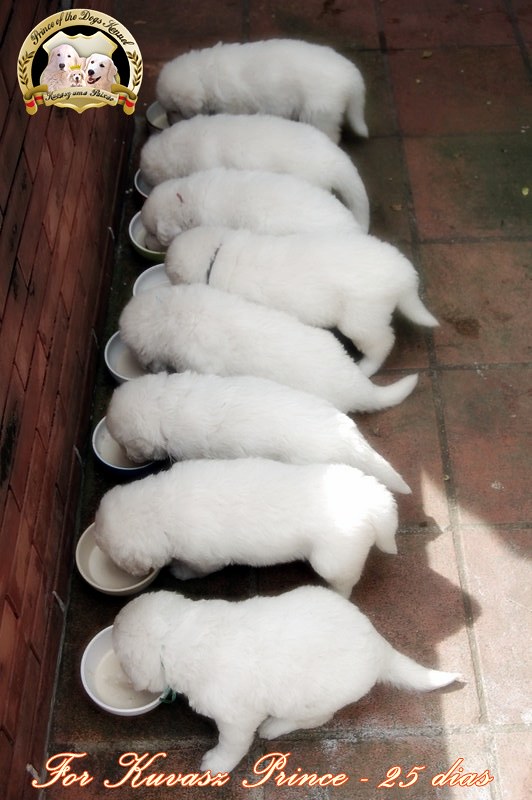The image showcases eight adorable, solid white puppies, each with short, stubby tails and black collars, eating from individual white bowls arranged in a row. They appear to be a few months old and are positioned on large red brick tiles next to a matching red brick wall. The photo is taken from a bottom-to-top perspective. At the bottom of the image, there is text in a non-English language that reads "four canvas prints, 25 dias." In the top left corner, there is a banner resembling a crest of arms featuring three white dogs and the word "Samantaba."